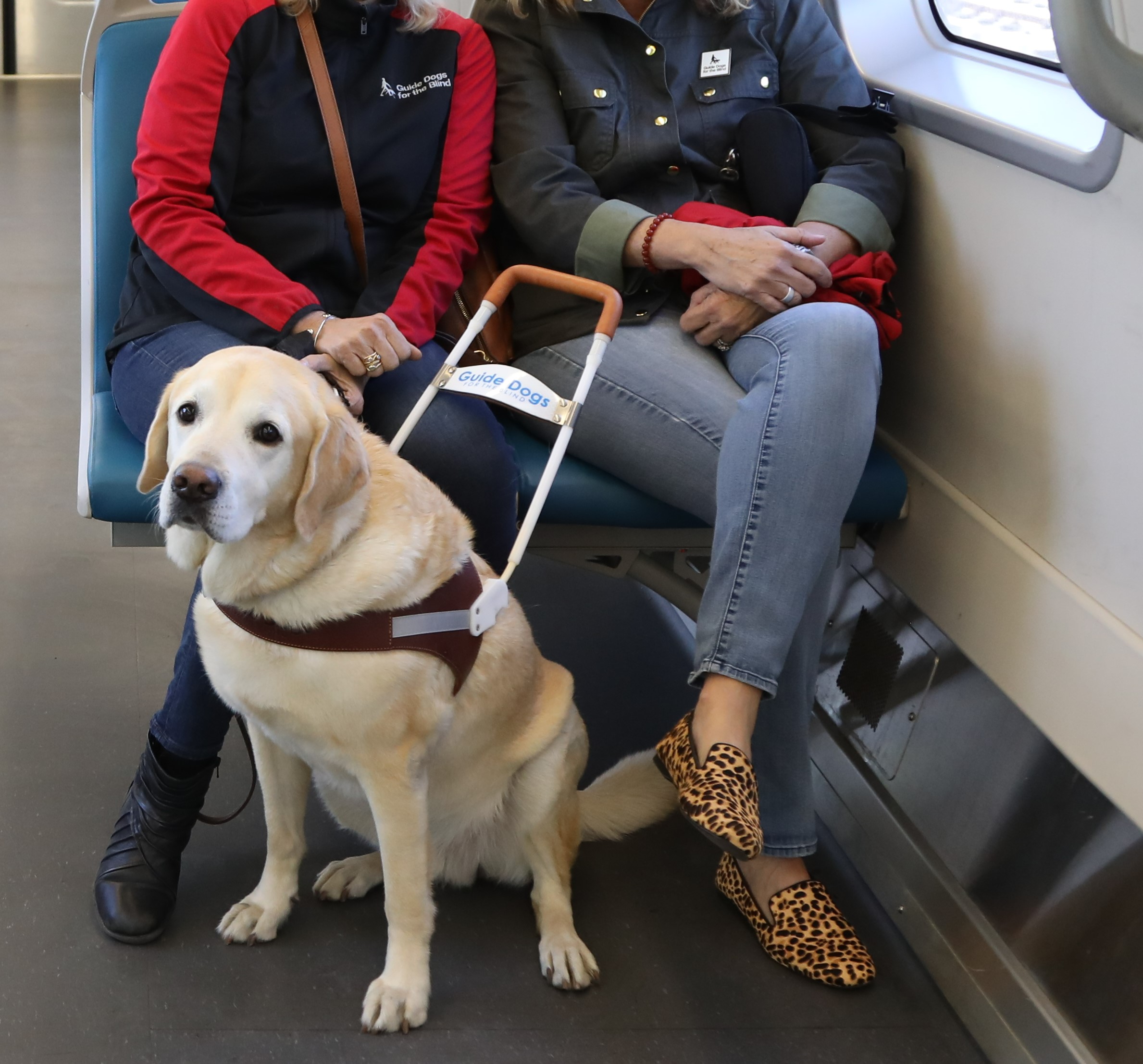This photograph captures two women seated on a blue bench aboard what appears to be a train or bus. Their upper bodies are out of frame, showing only from the neck down. Both are dressed in blue jeans. The woman on the left wears a navy jacket with red stripes down the sleeves and the words "Guide Dogs for the Blind" printed on it, while the woman on the right is in a dark blue jacket and orange cheetah-print loafers. In front of them sits a yellow Labrador or Labrador mix, a service dog. The dog, appearing older and somber, wears a distinctive harness with the label "Guide Dogs" on the handle, indicating its role as a guide for individuals who are blind or visually impaired. The dog's cream-colored fur and dignified presence add a touching element to this scene of companionship and assistance.